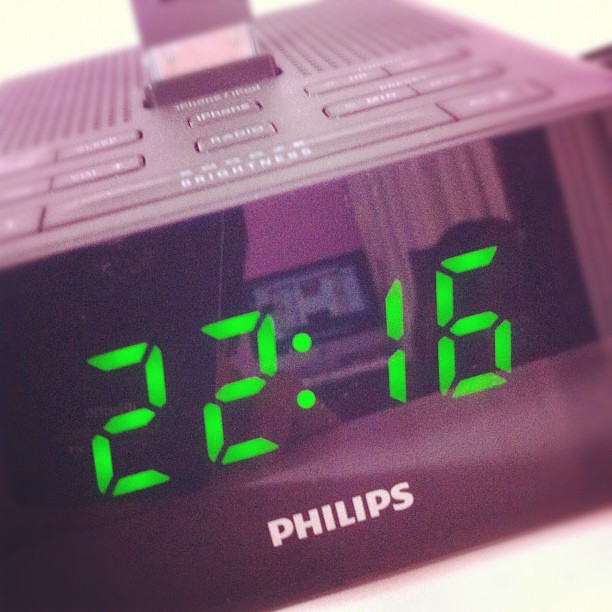The image features a Philips alarm clock, prominently displayed with a close-up view of its face. The clock itself is black, with the brand logo "Philips" printed in white at the bottom. The digital display shows the time as 22:16 in luminous green numbers. On the top of the clock, there are several buttons: a long brightness adjustment button, flanked by a 'radio' button on one side and an 'iPhone' button on the other. To the left of the brightness button are volume control buttons and a sleep button. To the right, there are min-max buttons and several other smaller, less discernible buttons. The device features speaker grilles with tiny holes on one side.

A reflection on the screen reveals part of a laptop in the background, though the content on the laptop is not visible. Additionally, the reflection captures a curtain and a portion of a wall, indicating that this scene is set in someone's room. The camera used to take the photo is also faintly visible in the reflection.